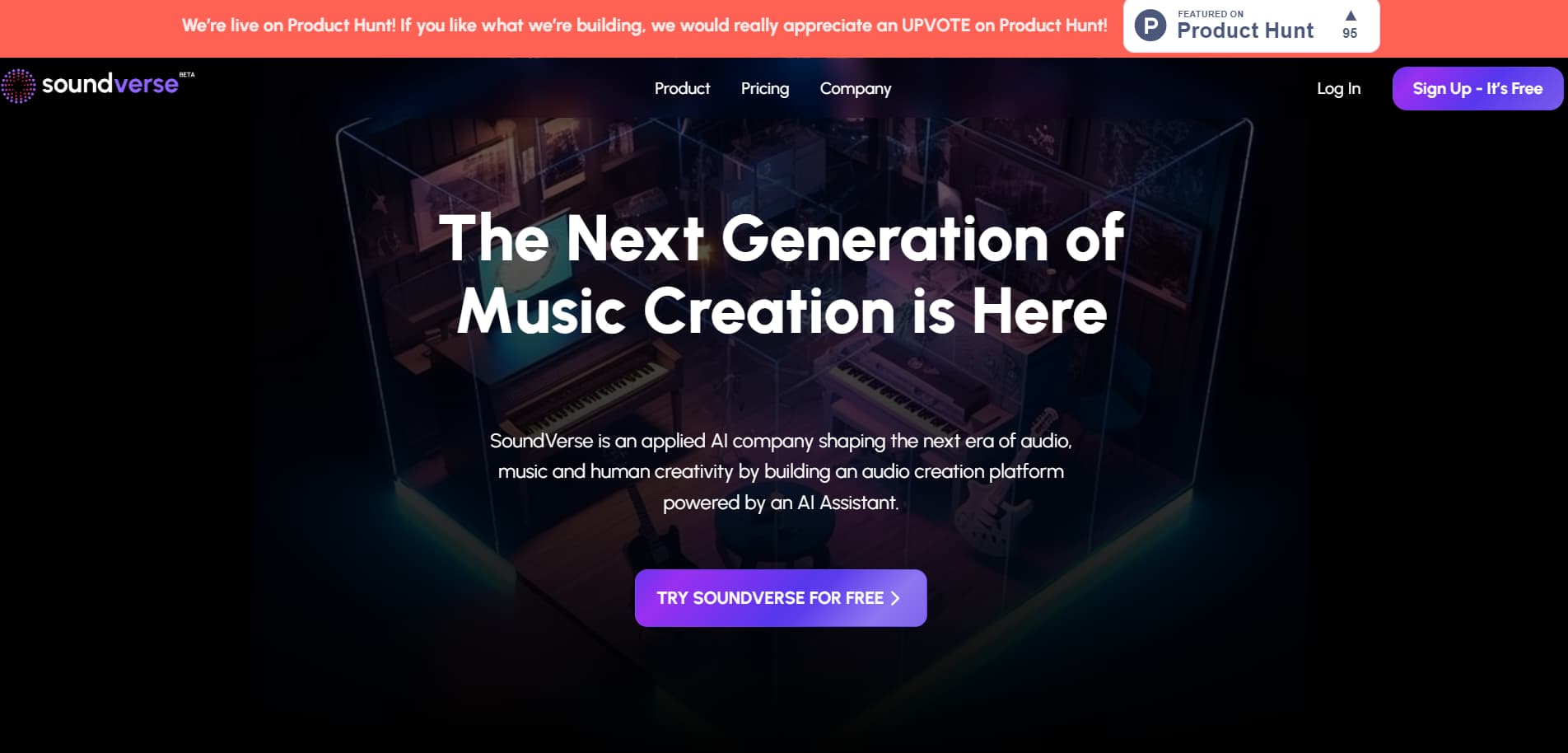The image depicts a website with a dark-themed design. In the top-left corner, the logo reads "SoundVerse," with "Sound" in white and "Verse" in purple. A prominent red bar at the top alerts users with the message "We're live on Product Hunt. If you like what we're building, we would really appreciate an upvote on Product Hunt," accompanied by a white box with "Product Hunt" written in black text.

The main section of the website features a very dark background with shades of purple, black, and gray. It portrays a studio-like environment with a transparent box containing a piano and several musical instruments, creating a somewhat enigmatic atmosphere.

Prominently displayed text states, "The Next Generation of Music Creation is Here." Further description introduces SoundVerse as "an applied AI company shaping the next era of audio, music, and human creativity by building an audio creation platform powered by AI."

At the bottom of the main section, a rounded purple bar invites users to "Try SoundVerse for Free," with an arrow pointing to the right, suggesting a call to action.